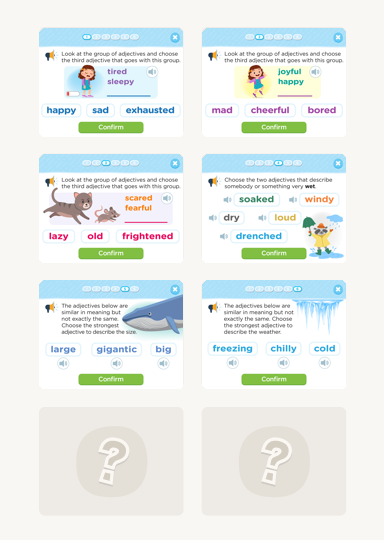This image depicts a vibrant and colorful educational website designed like an interactive quiz, possibly aimed at children. The website is structured into eight distinct sections, each resembling a comic-style card. Each card presents a group of adjectives and instructs the user to select the third adjective that fits within the group. 

For example, one card displays an illustration of a tired and sleepy girl with the adjectives "happy," "dead," and "exhausted" as choices, and includes a green "Confirm" button. Another card, with a similar instruction, shows the adjectives "joyful" and "happy," offering "mad," "cheerful," and "bored" as options, also featuring a green "Confirm" button.

Among the cards, one portrays an animal—perhaps a cat chasing a mouse—with the context "scared." It asks the user to pick the appropriate adjective from "lazy," "old," and "frightened." Each card is intricately designed with various vibrant colors, making the interface appealing and engaging for children.

Additionally, the image includes two cards towards the bottom with illustrations of a whale and water. Two more sections at the bottom remain undeveloped, depicted as gray circles with white-outlined question marks inside gray squares.